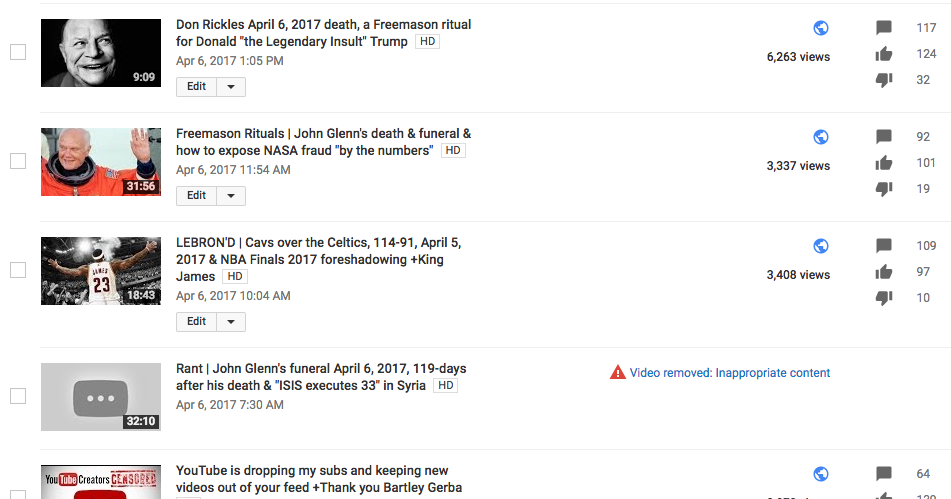**Detailed Descriptive Caption:**

The image is a detailed screenshot displaying the internal metrics and analytics of a YouTube channel, focusing on the performance of five specific videos. Each video is organized in its respective row, presenting crucial data such as views, comments, likes, and dislikes.

1. The top video is titled "Dawn Rickles April 6, 2017 Death: A Freemason Ritual for Donald 'The Legendary Insult Trump' HD." It was uploaded on April 6, 2017, at 1:05 p.m. The video has a black background and has accrued 6,263 views, 117 comments, 124 likes, and 32 dislikes.

2. The second video, "Freemason Rituals: John Glenn's Death and Funeral and How to Expose NASA Fraud by the Numbers Issue," was uploaded on April 6, 2017, at 11:54 a.m. This video has garnered 3,337 views, 92 comments, 101 likes, and 19 dislikes.

3. The third video, under the title "LeBron, Cavs Over the Celtics 114-91 April 5, 2017: NBA Finals 2017 Foreshadowing plus King James," was uploaded on April 5, 2017. It has obtained 3,408 views, 109 comments, 97 likes, and 10 dislikes.

4. Below that is a video titled "Rants: John Glenn’s Funeral April 6, 2017 - 119 Days After His Death." This video discusses the timeline of events following John Glenn’s passing. The exact metrics for this video are not fully detailed in the available information.

5. The final video mentioned, "Isis Executes 33 in Syria," seems to cover a significant and grim event. Again, the specific views, comments, likes, and dislikes for this video are not completely provided.

The screenshot offers an insightful look into the statistical performance and content themes present on this YouTube channel, illustrating a mixture of conspiracy theories, sports foresight, and real-world events as captured through the uploaded videos.